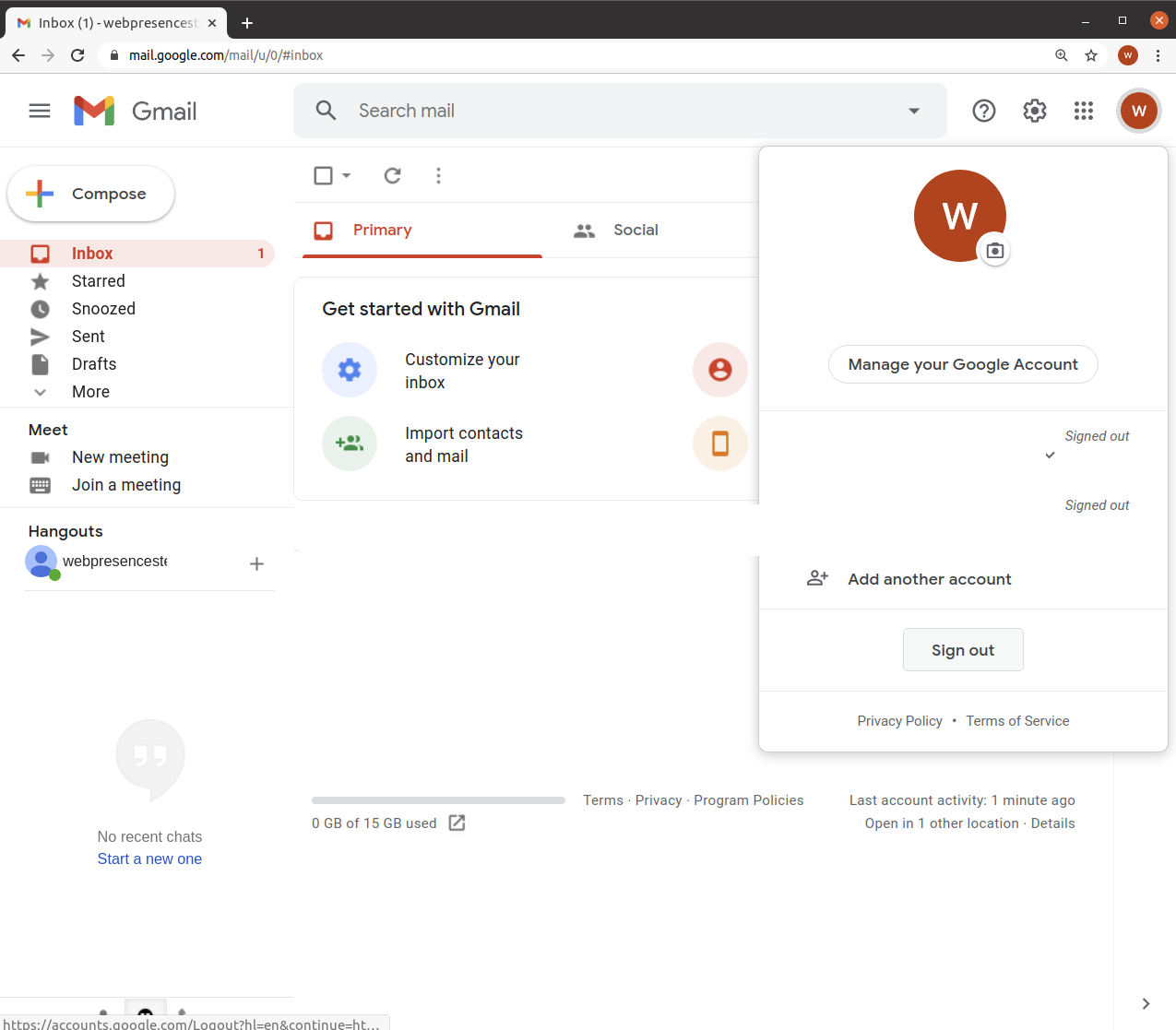A detailed screenshot of a Gmail inbox on a computer monitor. In the upper left corner, three horizontal bars, commonly referred to as a hamburger menu, allow access to additional navigation options. To their right is the multicolored Gmail "M" logo, with the word "Gmail" prominently displayed beside it. Moving further to the right, there's a search box ready to accept queries, identifiable by a magnifying glass icon on its left. Adjacent to this search box, icons for help (a question mark), settings (a gear), app selection (a grid of small squares), and user information (a red circle with a white "W" initial inside) are aligned.

On the left-hand side of the inbox, the familiar Gmail folders and functions are listed vertically: "Compose," "Inbox," "Starred," "Snoozed," "Sent," "Drafts," "More," and below them options for "New Meeting," "Join a Meeting," and "Hangouts." Next to "Hangouts," a notification green dot and the label "Web Presences" indicate recent activity.

In the central pane, the Inbox is selected and highlighted in red, displaying the "Primary" tab. A new email notification is visible, titled "Get started with Gmail," followed by prompts to "Customize your inbox" and "Import contacts and mail."

At the top right of the screen, the red circle with the white "W" is repeated, denoting the user's profile. Below it, a bar in black provides the option to "Manage your Google Account," showing that the user has a signed-out session indication active. Further options include a person icon with a plus sign to "Add another account," a gray box for "Sign out," and links to the "Privacy Policy" and "Terms of Service" at the bottom of the screen.